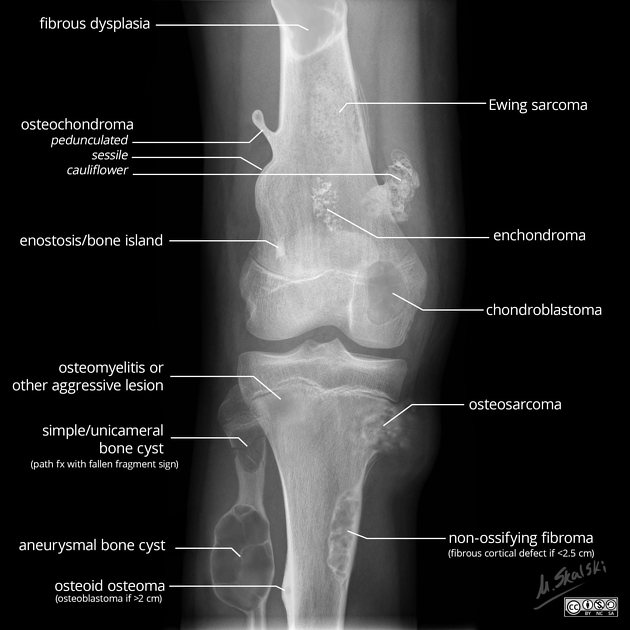This image features a detailed x-ray scan against a solid black background, capturing the intricate structure of a bone joint—likely the knee or elbow. The limb appears in various shades of gray, highlighting the bone in bright white. Numerous white lines with labels denote various bone conditions, including Fibrous Dysplasia, Ewing's Sarcoma, Osteochondroma, Pedunculated Sessile Cauliflower, Bone Island, Osteomyelitis or other aggressive lesions, Simple Unicameral Bone Cyst, Aneurysmal Bone Cyst, Chondroblastoma, Enchondroma, Osteosarcoma, Non-Ossifying Fibroma, Fibrous Cortical Defect (less than 2.5 cm), and Osteoid Osteoma. These labels, pointing to different spots on the bone, identify potential pathologies that could afflict the joint. In the lower right corner, a signature by M. Skalsky and a tiny, unidentifiable copyright logo further authenticate the image. The array of labels suggests a comprehensive examination documenting various possible bone diseases and abnormalities.